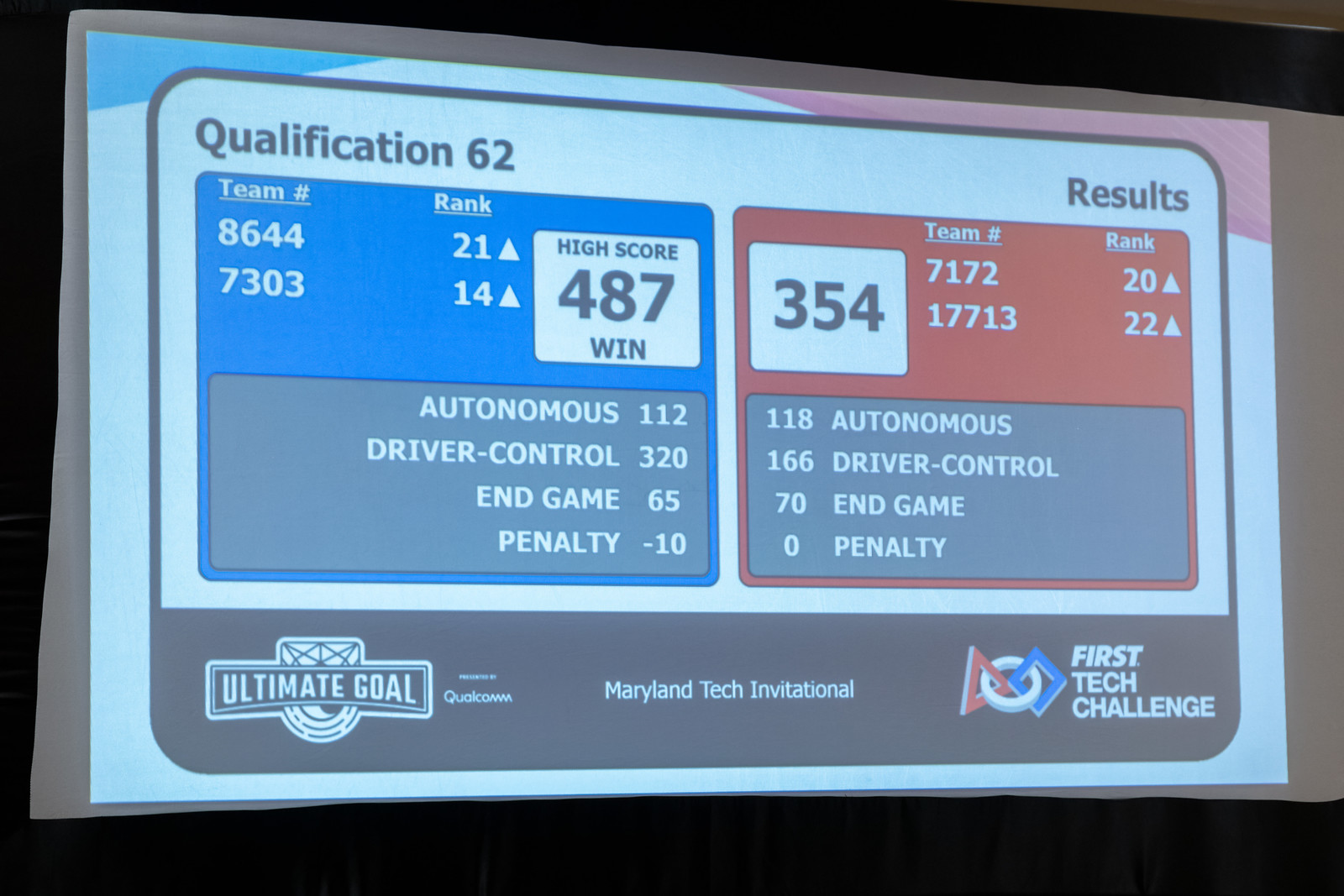The image is a photograph of a screen displaying the results of a game at the Maryland Tech Invitational, part of the First Tech Challenge. The screen has a rectangular shape with a black and white boundary, and the photograph is slightly faded as it was taken through the screen. At the top left corner, it says "Qualification 62," and on the right, "Results." Two sections on the screen represent two teams: blue and red. The blue team, consisting of Team 8644 ranked 21st and Team 7303 ranked 14th, won with a score of 487, broken down as follows: Autonomous 112, Driver Control 320, End Game 65, and a Penalty of -10. The red team, consisting of Team 7172 ranked 20th and Team 17713 ranked 22nd, scored 354 with components: Autonomous 118, Driver Control 166, End Game 70, and no penalties. At the bottom of the screen, the logos and text indicate the event is part of the "Ultimate Goal" challenge, presented by Qualcomm, with titles "Maryland Tech Invitational" and "First Tech Challenge."